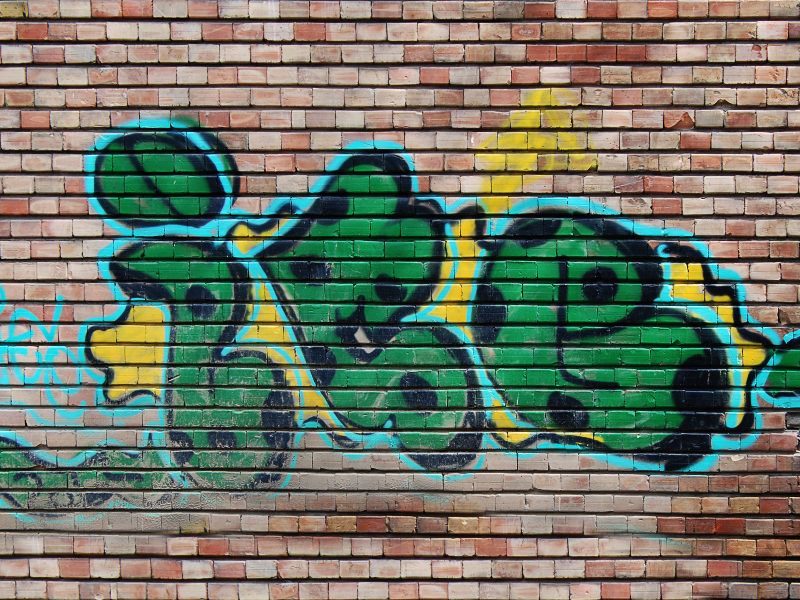The image captures vibrant graffiti on a worn, flat-looking red brick wall with black mortar joints. Dominating the wall are stylized green letters, "I-R-G," adorned with black polka dots and outlined in black. These eye-catching letters are encased in a blue border. A yellow banner with black squiggle marks serves as the backdrop for the letters, adding contrast and depth. Notably, the "I" is creatively depicted as a snake with a curvy body extending towards it. The photograph cuts off additional graffiti on this striking mural, hinting at more artwork beyond the frame. The wall, though primarily red brick, features some faded, whitish-beige patches, adding texture and emphasizing the urban setting.